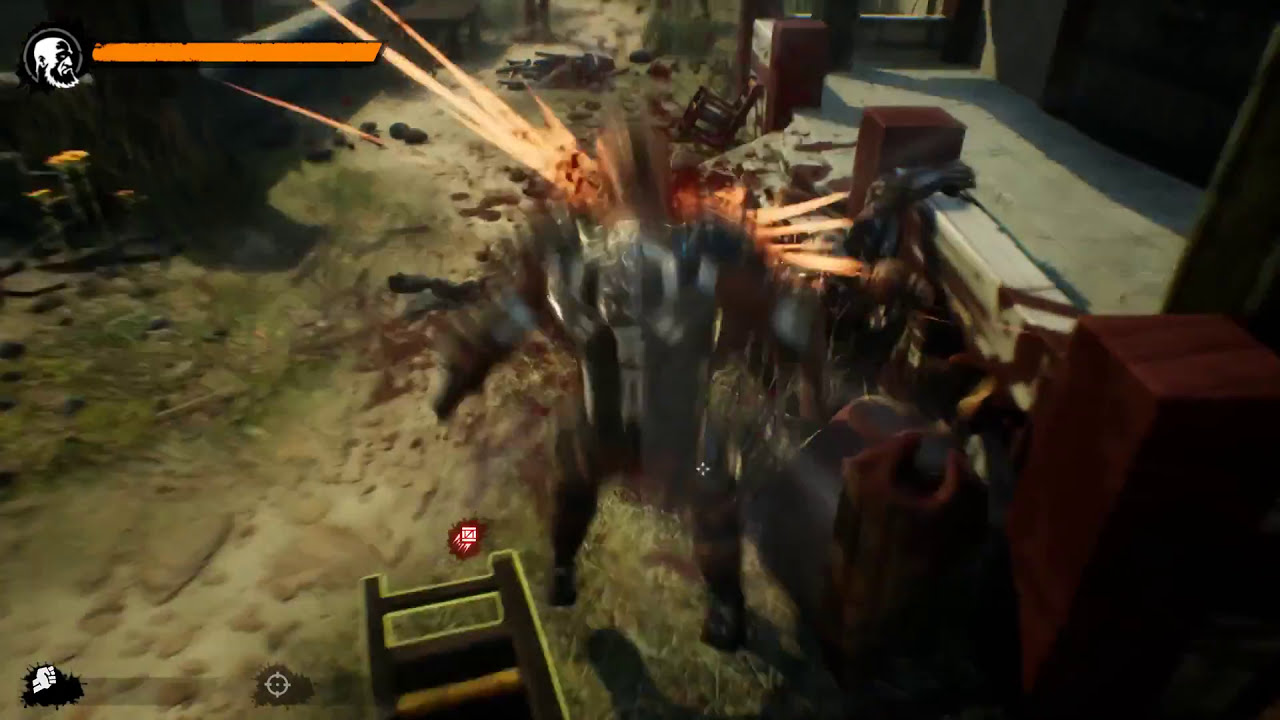In this image, we see a detailed screenshot from a 3D video game, characterized by a chaotic and action-packed scene. At the forefront is a heavily armored character, whose distinctive features include a blurred, rapidly moving head—possibly indicating a mohawk—and steel plates on their arms and chest. This blurriness suggests high-speed motion, potentially from an explosion visible with orangish-yellow lines and scattered debris around the character. The ground is a mix of grass and a dirt path with stone walkways, and in the environment, there are wooden posts, a building with a garage-like entrance, and nearby structures featuring a porch with red pillars leading to a concrete floor. Dead characters can be seen ahead along the path. The upper left corner displays an orange health bar and a black-and-white avatar face, indicating the game’s HUD.